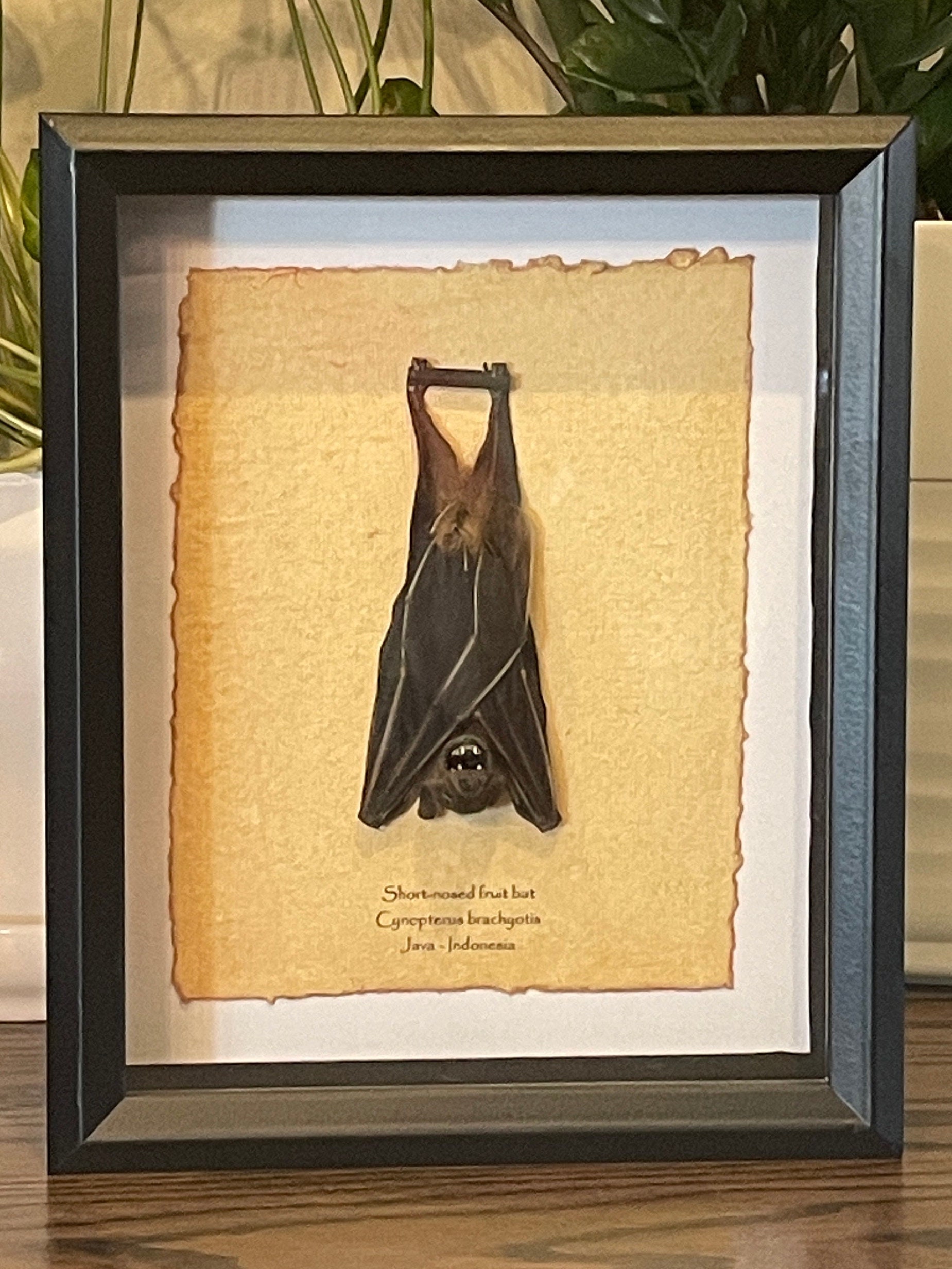This image showcases a framed, artistic depiction of a short-nosed true bat (Cynopterus brachyotis) from Java, Indonesia. The bat, drawn in striking black detail, is hanging upside down from a small brown rod, with its feet gripping each end of the rod. The bat's wings are folded over its body, exposing its head and open mouth, revealing white teeth. This illustration is set against a yellowish-brown piece of parchment paper, which is mounted on a white mat within a dark wooden frame. Below the bat's image are three lines of black text, though the exact wording is not clearly visible. The frame rests on a shiny wooden surface, possibly a tabletop, and the background of the photo is largely obscured by the frame, although some hints of a white wall and plants can be seen. The overall presentation resembles a scientific display, highlighting the bat as the main focus amidst the understated surroundings.